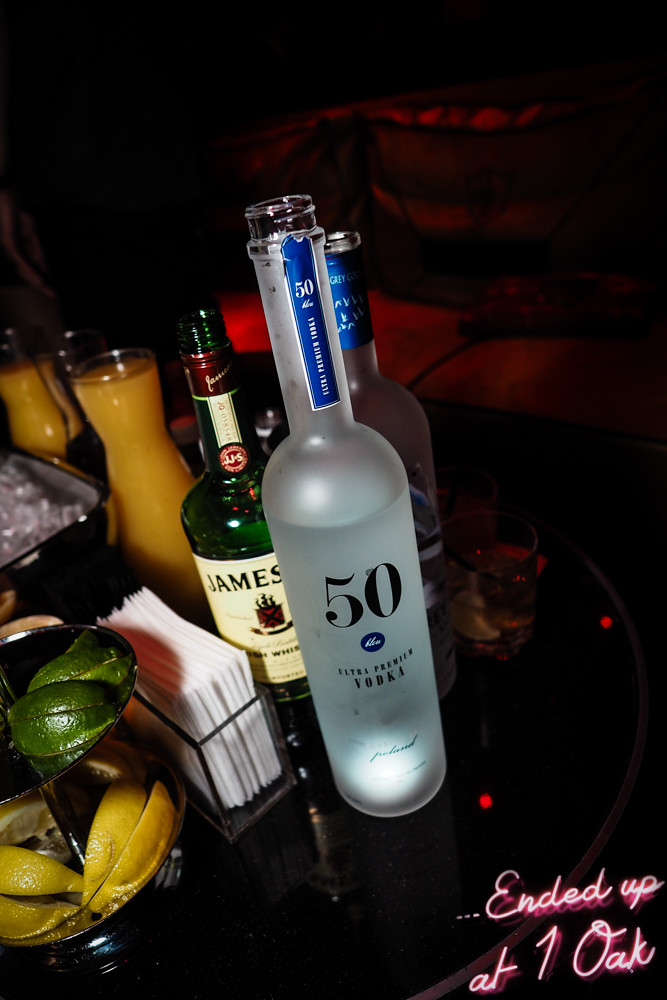This photograph, taken with a flash in a dimly lit nightclub or bar, captures a detailed scene atop a black bar table. The dark surroundings are punctuated by red lighting in the upper right, suggesting a nearby seating area, possibly cushioned couches. On the table, there is a small silver dish containing neatly cut lime and lemon wedges, alongside a napkin holder filled with white napkins. Prominently displayed are several liquor bottles, including a tall open bottle of Grey Goose vodka with a number 50 on it and a green bottle of Jameson whiskey with a light-colored label. Behind these, almost to the top, are two carafes filled with orange juice. Additionally, there's a small ice bucket visible on the bar top. In the lower right-hand corner of the image, written in neon pink, is the phrase, "...ended up at One Oak," suggesting the location of the photograph, likely a well-known bar or lounge.